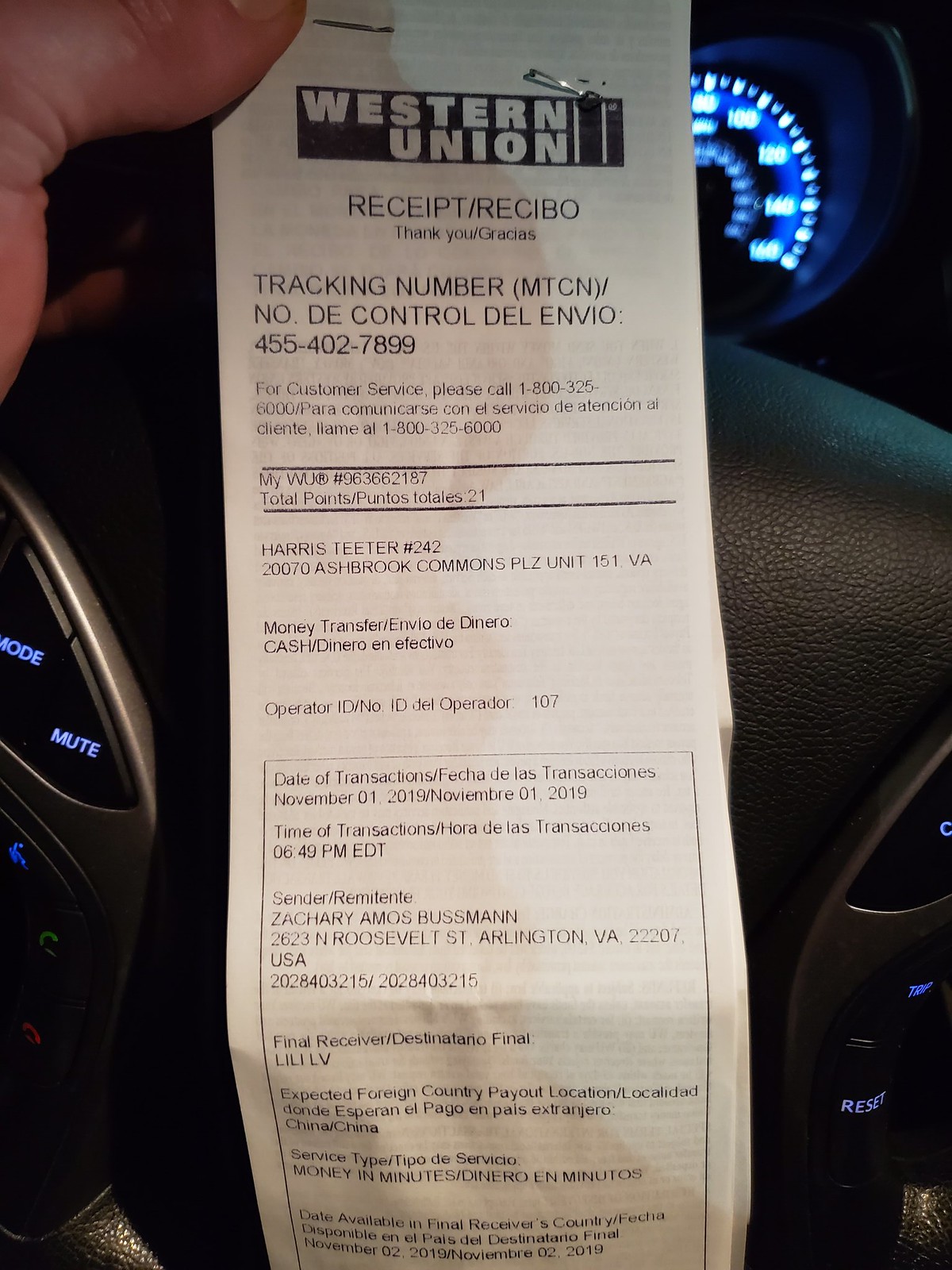This detailed caption describes an image of a Western Union receipt, captured inside a car at night. The receipt, featuring black text on white paper, prominently displays the Western Union logo at the top with contrasting white lettering. It contains bilingual elements, including phrases like "Thank you" and "Gracias," as well as "Receipo." The receipt includes critical information such as a tracking number, total points amounting to 21, customer service details, operator number, and a timestamp of 6:49 p.m. on November 1st, 2019. The photograph is taken inside a vehicle, with the dark background illuminated by the car’s dashboard lights, which shine in bright electric blue hues. The receipt is held up in front of the car's speedometer, indicating the vehicle might be an American make.